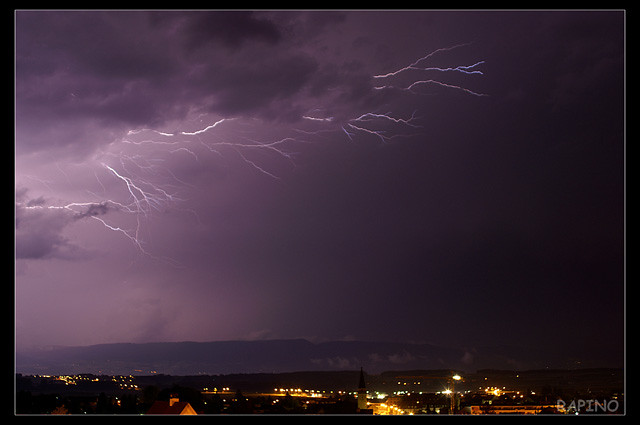A striking photograph captures a dramatic nighttime storm. On the left side, multiple vivid lightning bolts illuminate dark gray clouds, casting a purple hue across the sky. The right side of the image fades to deep black, emphasizing the intensity of the storm. Below, in the distance, a faint mountain range adds depth to the scene, while closer, an urban setting with various roads and twinkling lights in shades of orange and yellow provides contrast. Encasing the photograph is a black frame with a thin white inner border, adding a formal touch. In the bottom right corner, a watermark reading "B-A-P-I-N-O" subtly marks the creator's presence.